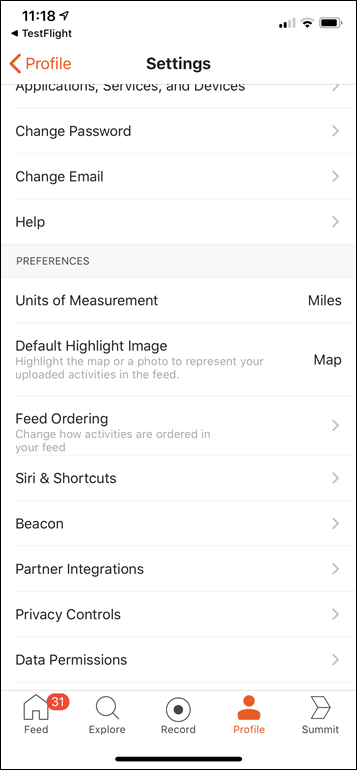This image is a detailed screenshot from an Apple iPhone, showcasing the settings page of a fitness tracking application running on the iOS operating system. The image has a clean, white background with predominantly black text, ensuring a stark contrast for readability. 

At the very top left of the screen, it displays the current time, 11:18 AM. Next to it, on the top right, icons reflect the phone's data and wireless signal strength, accompanied by a nearly full battery icon. 

Centered at the top of the image, in bold black text, is the word "Settings." To the left, in orange text, is the word "Profile" with an adjacent orange arrow pointing left, indicating navigation back to the profile page within the app.

The main content consists of several rows of settings options, each clearly labeled. These include "Change Password," "Help," "Units of Measurement," "Feed Ordering," "Beacon," "Privacy Controls," among others, suggesting that this app is designed for fitness or activity tracking. The presence of options like "Units of Measurement" and "Beacon" further supports its usage for tracking physical activities, in line with apps such as Strava.

At the bottom of the screen, there are five icons representing different sections of the app. These are, from left to right: "Feed," which includes an orange circle with the white number 31, indicating notifications or updates; "Explore"; "Record"; "Profile," which is highlighted in orange, signaling it as the current active tab; and "Summit."

This detailed layout provides a comprehensive overview of the app's settings page, illustrating a user-friendly and functionally rich fitness tracking application on an iPhone.